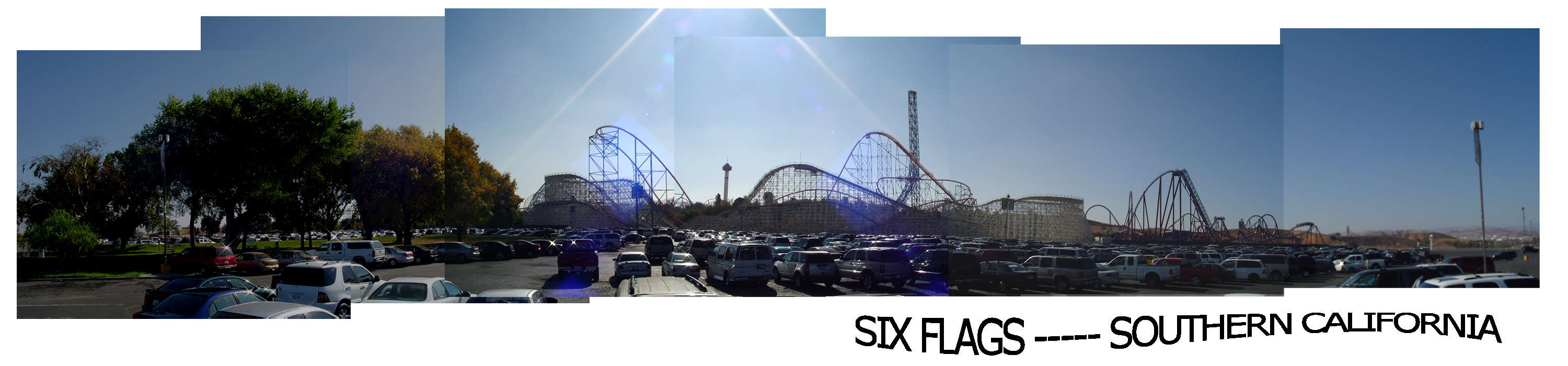This advertisement for Six Flags, Southern California, features a composite image composed of six overlapping pictures arranged horizontally to create a panoramic view. The image captures a vibrant scene of the amusement park, with lush green trees on the left transitioning to an array of roller coasters and other rides set against a clear blue sky. In the foreground, a bustling parking lot filled with cars in various colors, including red, white, and blue, is clearly visible. Sunlight streaks down through the center of the image, forming a triangular beam of light that adds to the dynamic atmosphere. The text, "Six Flags, Southern California," is prominently displayed in black at the bottom right corner of the image. The entire composition presents an enticing and lively snapshot of the amusement park, inviting visitors to explore and enjoy the attractions.